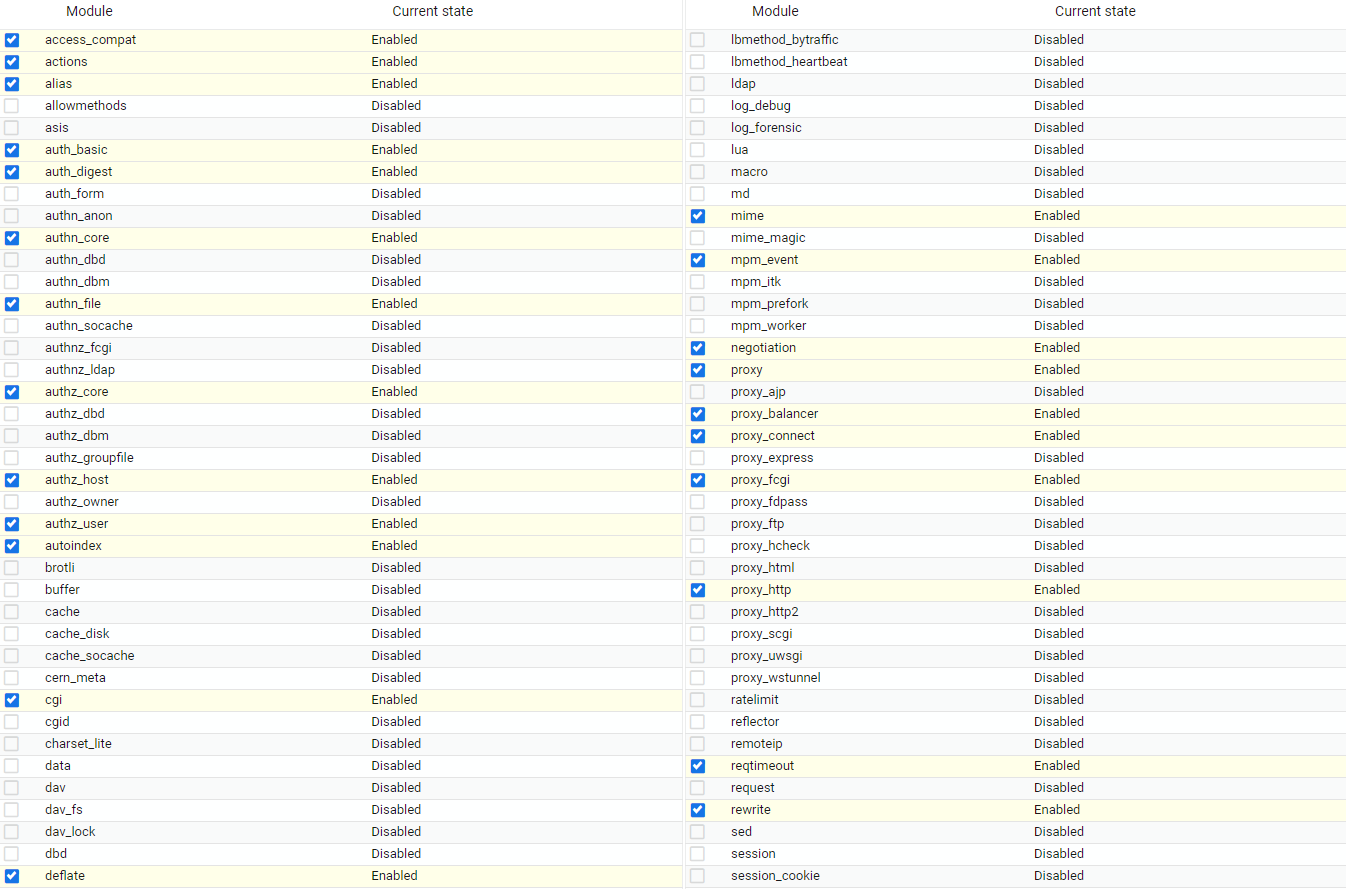The document contains a detailed table with multiple columns and rows. On the far left side of the table, there are checkboxes; some filled with a blue background and a white checkmark, while others remain empty. Adjacent to these checkboxes, the column titled "Module" lists various modules such as "access," "compat," "actions," "alas," and "allow methods." 

Next to the "Module" column, another column labeled "Current State" indicates whether each module is either "enabled" or "disabled."

In a mirrored layout, the table extends with another set of checkboxes on the left. Again, some of these are filled with a blue background and a white checkmark, while others are left blank. The subsequent "Module" column features entries like "macro," "MD," "mime," "proxy FTP," "proxy HTTP," and "request." Immediately following, the "Current State" column reflects the status of each module, signifying "disabled" or "enabled."

Each row is uniquely colored, alternating between blue, yellow, white, and gray, providing visual distinction. All the text within the table is rendered in small black print.